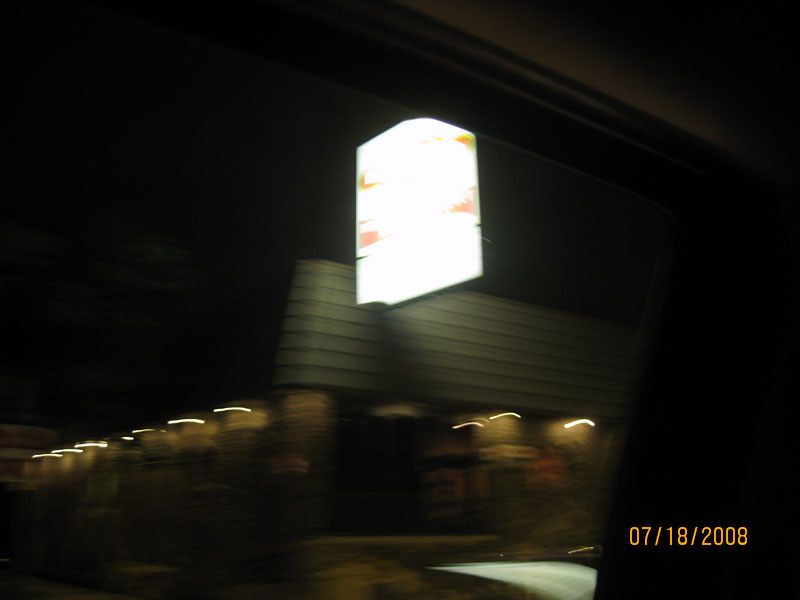A floating white square is prominently featured against a backdrop of gray paneling. Several linear streaks of yellow lights span from the left side of the image, indicating camera movement. The scene includes a grayish roof with intricate pipework. At the bottom left, a trash can sits near a dark, black door. In the bottom right corner, the date "07/18/2008" is displayed in a yellowish-orange hue. A sign is visible on the corner of the image, adding to the urban, industrial atmosphere.